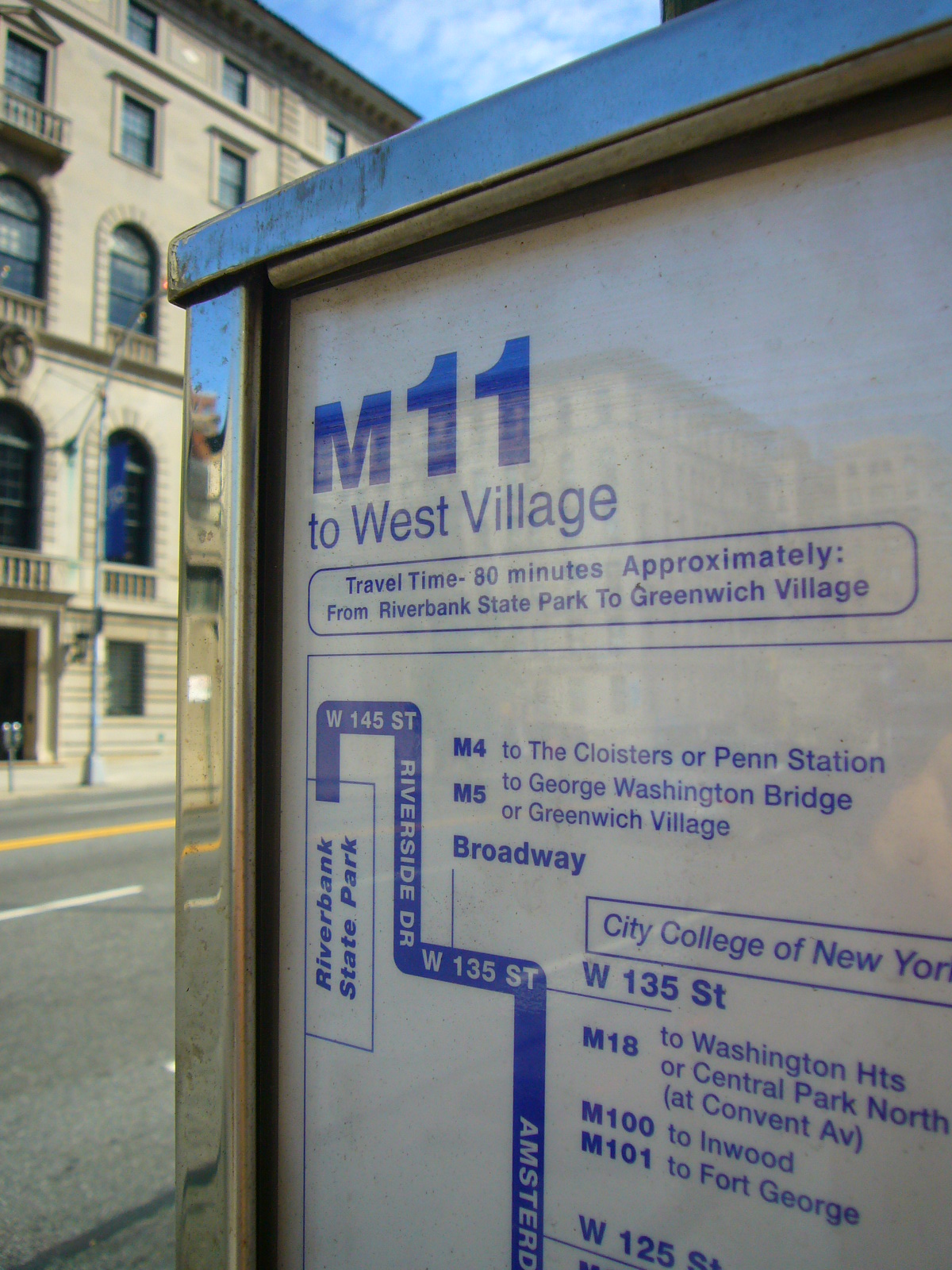The image depicts an outdoor scene featuring a street sign enclosed in a glass and metal frame. The sign, situated to the right, has a white background with blue text prominently displaying "M11 to West Village." Below, it states, "Travel time 80 minutes approximately from Riverbank State Park to Greenwich Village." The sign includes a detailed map outlining various transit routes and stops. Key points on the map list "Riverbank State Park," "M4 to the Cloisters or Penn Station," and "M5 to George Washington Bridge or Greenwich Village." Additionally, it points to "Broadway" and mentions "City College of New York" and "West 135th Street." Further down, it indicates connections to "M18 to Washington Heights or Central Park North at Convent Ave," "M100 to Inwood," and "M101 to Fort George." To the left of the sign, there are multiple roads and a building with five stories, featuring a light pole reaching up to the second floor. The scene also includes part of a blue sky with clouds above.